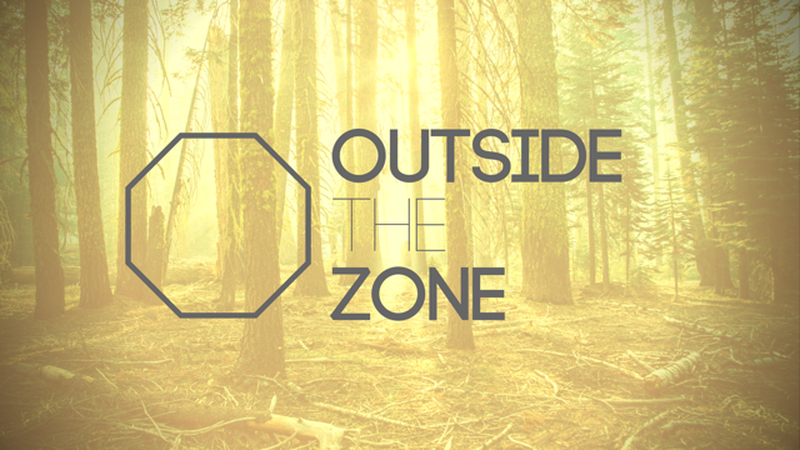The image displays a picturesque outdoor scene, tinted with a yellowish hue, set in a forest with an array of tall tree trunks, some crowned with branches and leaves. The background shows a faint, sunlit forest creating a serene atmosphere. The forest floor is littered with scattered branches, sticks, and dirt, presenting a rugged, earthy brown texture. Central to the image is a logo and text composition. On the left side, there's a blue-outlined octagon reminiscent of a stop sign, unfilled. To its right, the words "outside the zone" are prominently displayed in blue, left-aligned but positioned in the middle of the frame. The phrase is stylized with "outside" and "zone" in a thicker font, contrasting with the thinner "the" nestled in between. The overall colors in the image range from brown, tan, and gray to subtle hints of green and blue, blending natural and designed elements harmoniously.